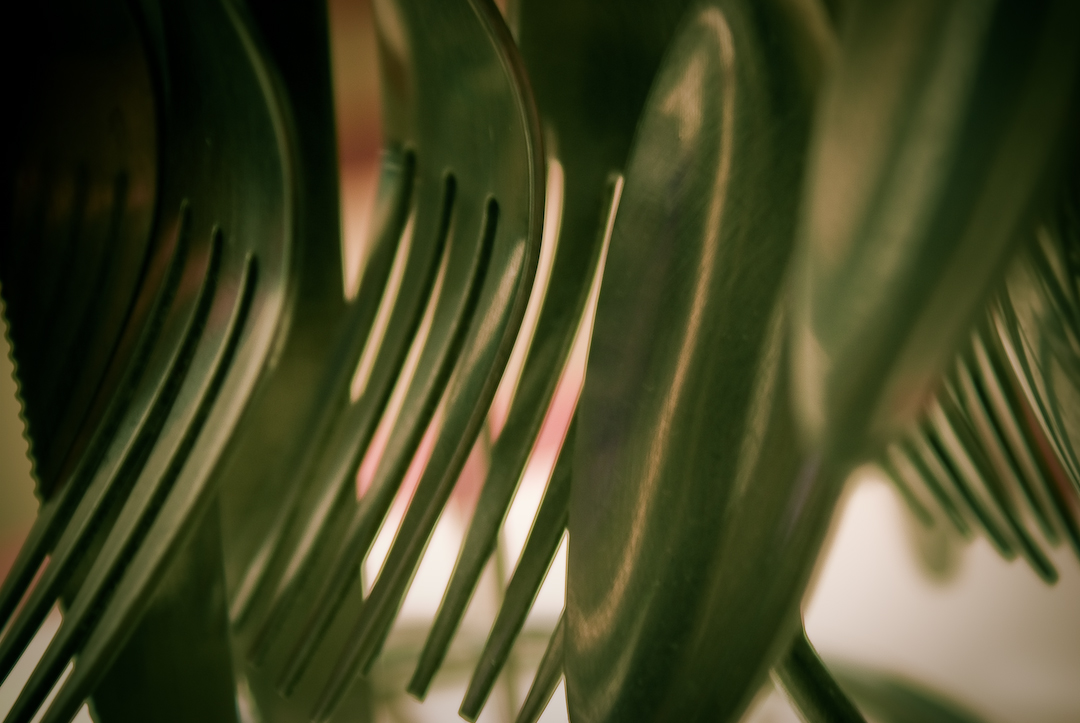The image captures an extremely close-up view of various cutlery, prominently featuring a multitude of silver, polished forks organized in several rows. Each fork has four tines, and there appear to be approximately a dozen or more of them densely arranged, making up the majority of the objects in the frame. The forks give the impression of either hanging from something or being arranged in a manner akin to being placed in a dishwasher, where only the fork heads are visible.

Interspersed among the forks are a few spoons, notably fewer in number compared to the forks. Specifically, two shiny silver spoons can be seen, adding some diversity to the arrangement but maintaining the reflective, polished appearance shared by all the utensils. There is also a single knife present in the composition. The tight framing of the photograph focuses solely on the utensil heads, with no handles visible, creating an abstract, almost plant-like visual effect upon initial viewing.

The background of the image is blurred, rendering the surrounding context indistinct and emphasizing the meticulous details of the cutlery. This blurring effect contributes to the ambiguity regarding whether the utensils are simply laid out or hanging. The polished surfaces of the utensils reflect light, adding to the image's highly detailed and shiny appearance.